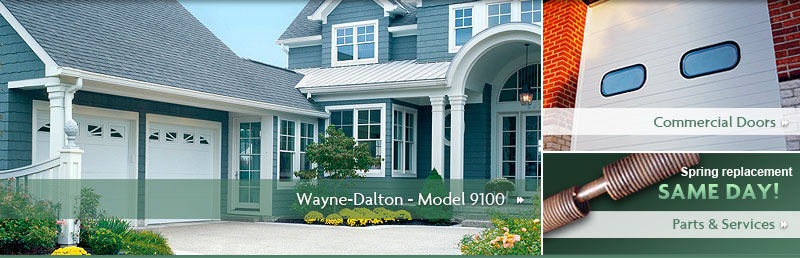This horizontally cropped screenshot features two side-by-side images. The left image, a large rectangular photo, partially displays the front view of a house with an attached garage situated vertically rather than on the side. A green banner at the bottom reads "Wayne Dalton Model 9100," with an arrow pointing to the right. The right image, a smaller square photo, is a split view. The top part shows a large commercial garage door affixed to a brick building, accompanied by a white banner across the bottom that says "Commercial Doors" in gray. Below, a smaller rectangle displays a slanted photo of a spring with the text "Spring Replacement Same Day." At the bottom, a white banner reads "Parts and Services," along with a play button on the right-hand side.